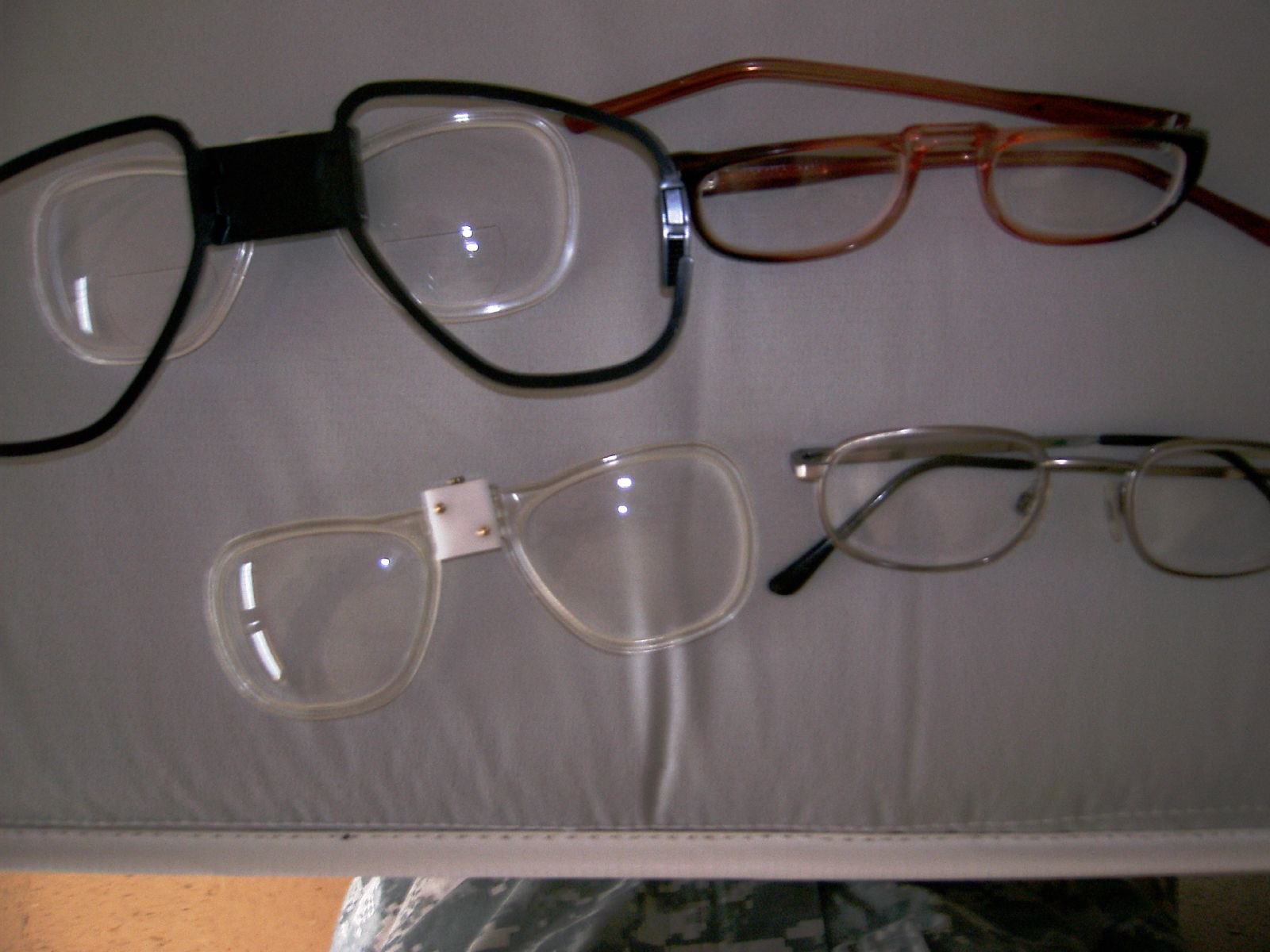This rectangular photograph presents a close-up view of five pairs of eyeglasses artfully arranged on a dark grey background. In the upper left corner, there is an oversized pair with a prominent dark black frame. Just inside the large lenses of the black glasses is a pair of smaller, clear-framed glasses featuring rounded lenses at the bottom. Adjacent to these glasses on the right is a pair with dark brown frames that fade into a lighter, opaque brown towards the arms, creating a distinctive gradient effect. Below these glasses are two more pairs positioned side by side. On the left, there is a set of clear plastic aviator-shaped glasses with a square bridge featuring two rivets at the nose piece. To the right of these is a pair with a sleek design: black coloring around the ends of the arms at the temples that transitions into a silver metal frame, neatly outlined in silver. The varying shapes, colors, and sizes of the eyewear create an intriguing visual ensemble.